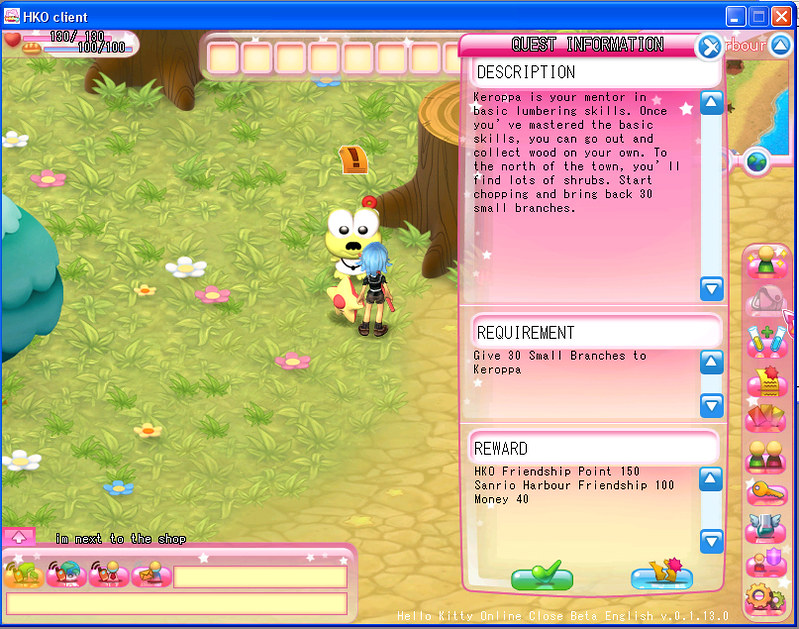This is a screenshot of a video game, displayed in a typical windowed application format on a PC with the title "HKO Client" at the top. In the outdoor scene, two characters are standing near the stump of a tree surrounded by grass and scattered pale pastel flowers in shades of white, pink with yellow centers, yellow with orange centers, and blue with yellow centers. To the left, the tip of a tree is visible. One character, a girl with blue hair, is facing away from the viewer, dressed in a black top, dark shorts, and dark shoes, holding a red staff in her right hand. She appears to be interacting with a mini dinosaur or dragon that is facing the viewer. This creature is yellow with pink dots, large eyes, a black nose, a small mouth, and a white collar. Above its head is a rectangle with an exclamation point. 

At the top of the screen, there's a blue edge with the text "HKO Client" and a number ticker in the left corner showing "100/130" with a heart icon and "100/100" next to a hot dog or mushroom-like symbol. On the right side of the screen, there is a rectangular section titled "Quest Information Description" that reads: "Caropa is your mentor in basic lumbering skills. Once you have mastered the basic skills, you can go out and collect wood on your own. To the north of the town, you will find lots of shrubs. Start chopping and bring back 30 small branches." Below this are smaller rectangles labeled "Requirement: Give 30 small branches to Caropa," and "Reward: HKO, Friendship point 150, Sanrio Harbor Friendship 100, Money 40." In the bottom left, there's a text box stating "I'm next to the shop," flanked by pink ticker tapes with various logos and caricatures on both sides of the screen.